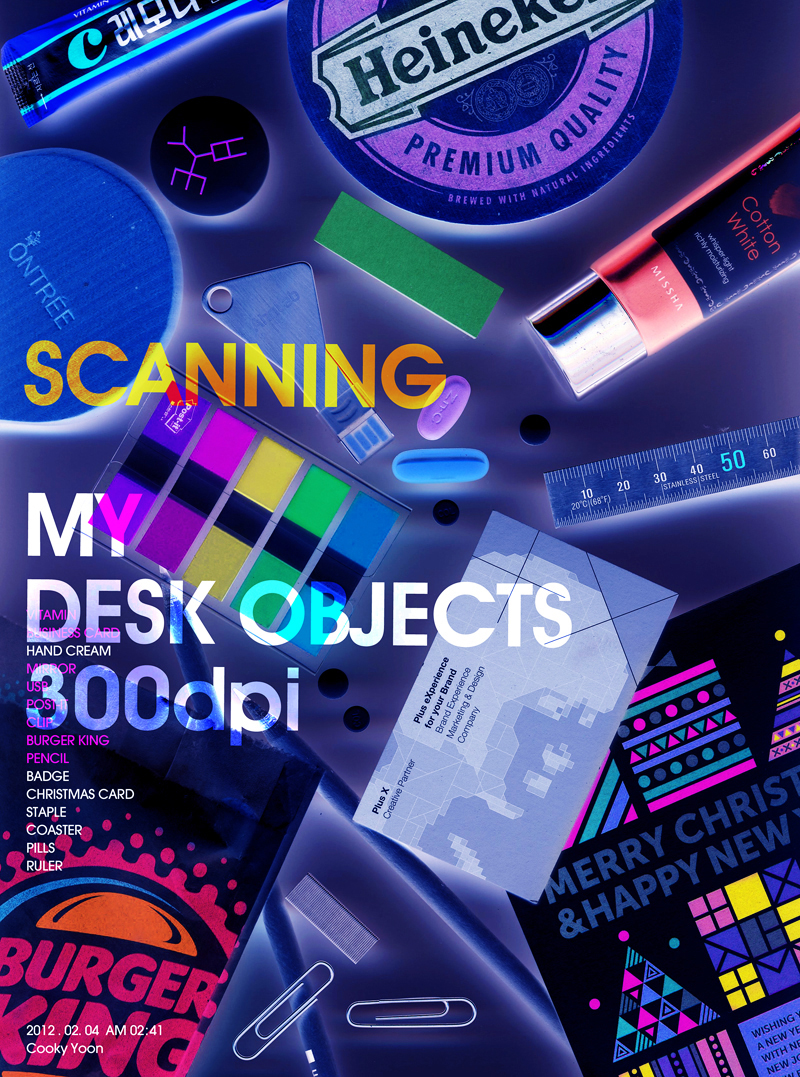The image is a detailed, color illustration resembling a magazine cover, presented in portrait orientation. It depicts a cluttered desktop with various objects meticulously illustrated and arranged on a dark blue surface. The composition is headlined with the text "Scanning My Desk Objects 300 DPI," with "Scanning" in gold typography and "My Desk Objects 300 DPI" in white, featuring some imagery visible through the lettering.

The illustrated objects are tightly packed and include a variety of common desk items. In the top right corner, there is a circular Heineken can seal, adjacent to a red tube of makeup, and below that, a ruler. Toward the bottom right is a modern graphic Christmas card partially visible, with the words "Merry Christmas and Happy New Year" partially cut off. At the bottom edge, two paper clips and a piece of staples are positioned beneath a business card.

In the bottom left corner, a brightly colored Burger King package stands out in pink and orange hues. Scattered among these items are additional objects such as a lip gloss tube, pills, a hand cream container, and five colorful tabs resembling those used in notebooks. The overall artistic style is modern, with a focus on detailed illustration. The background imagery supports the notion that these are typical desk objects, fitting the title’s theme of scanning one’s desk at 300 DPI.